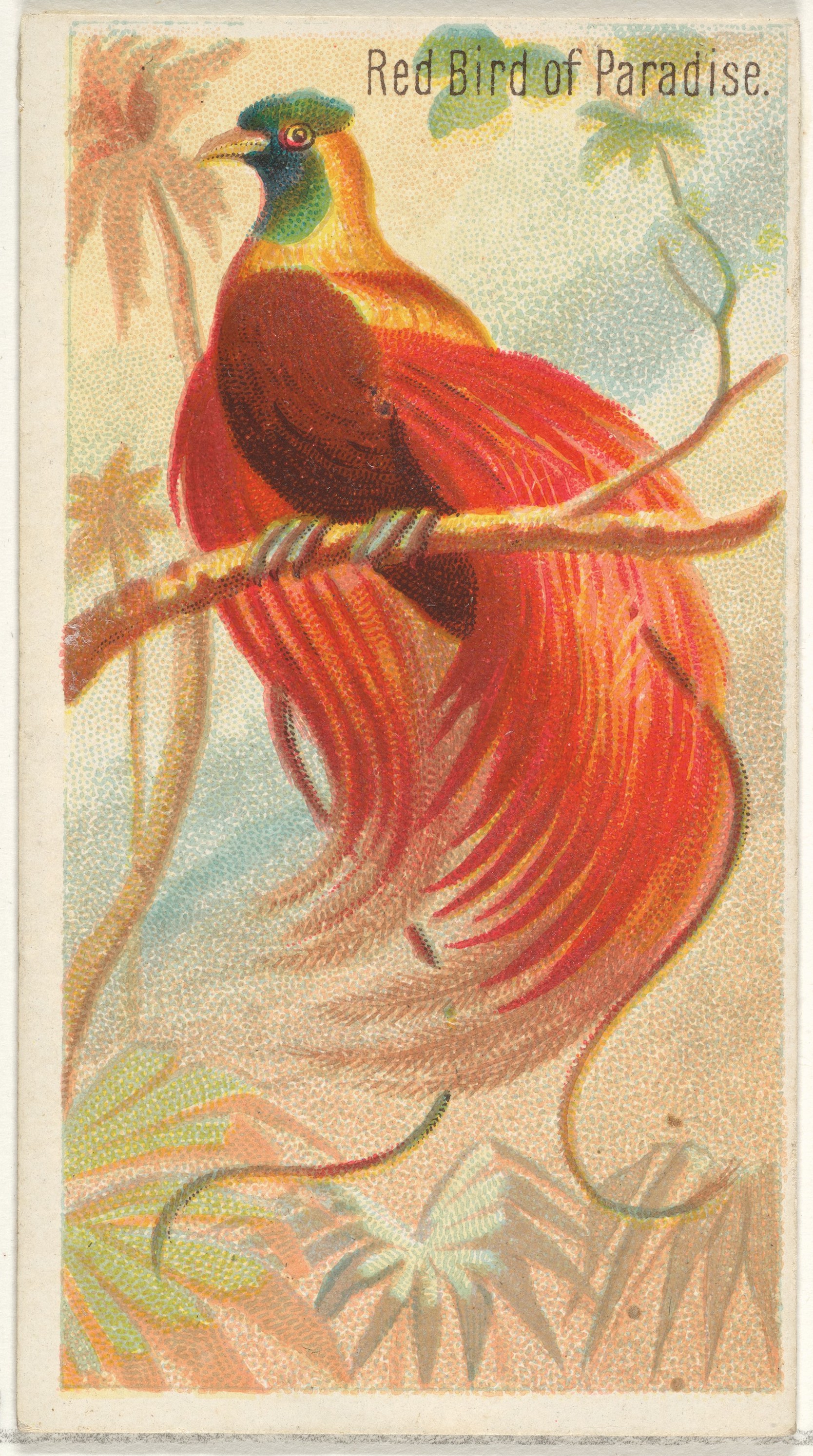This image showcases an intricate drawing of a red bird of paradise, prominently placed as the main focal point. The bird, with its splendid and extensive plumage of bright red and maroon feathers, elegantly extends past a slender tree branch it is perched on with its three-fingered claws. The bird’s intricate coloration features a dark red chest, and wings that transition to a lighter red with streaks of yellow, blending into a mustard-yellow and golden-orange back. Its head is adorned with a teal-green or blue-green hue, including similar coloring under its eyes, and is accented with a small, sharp tan beak.

The drawing also displays a vibrant setting, complemented by a detailed background. Near the bird’s beak, a red flower with a lengthy brown stem appears to be within reach, adding to the visual interest. Additional green flowers embellish various parts of the image, particularly in the upper right and bottom sections. Enhanced by a textured, potentially yellowed backdrop, palm trees in shades of red further enrich the scene on the left side. The overall composition suggests a stylized approach with patterned leaves at the base and the prominent text "red bird of paradise" emblazoned in the top right corner, affirming the species depicted. The artwork likely resides on what appears to be a textured canvas or scroll, giving it a timeless and tactile quality.